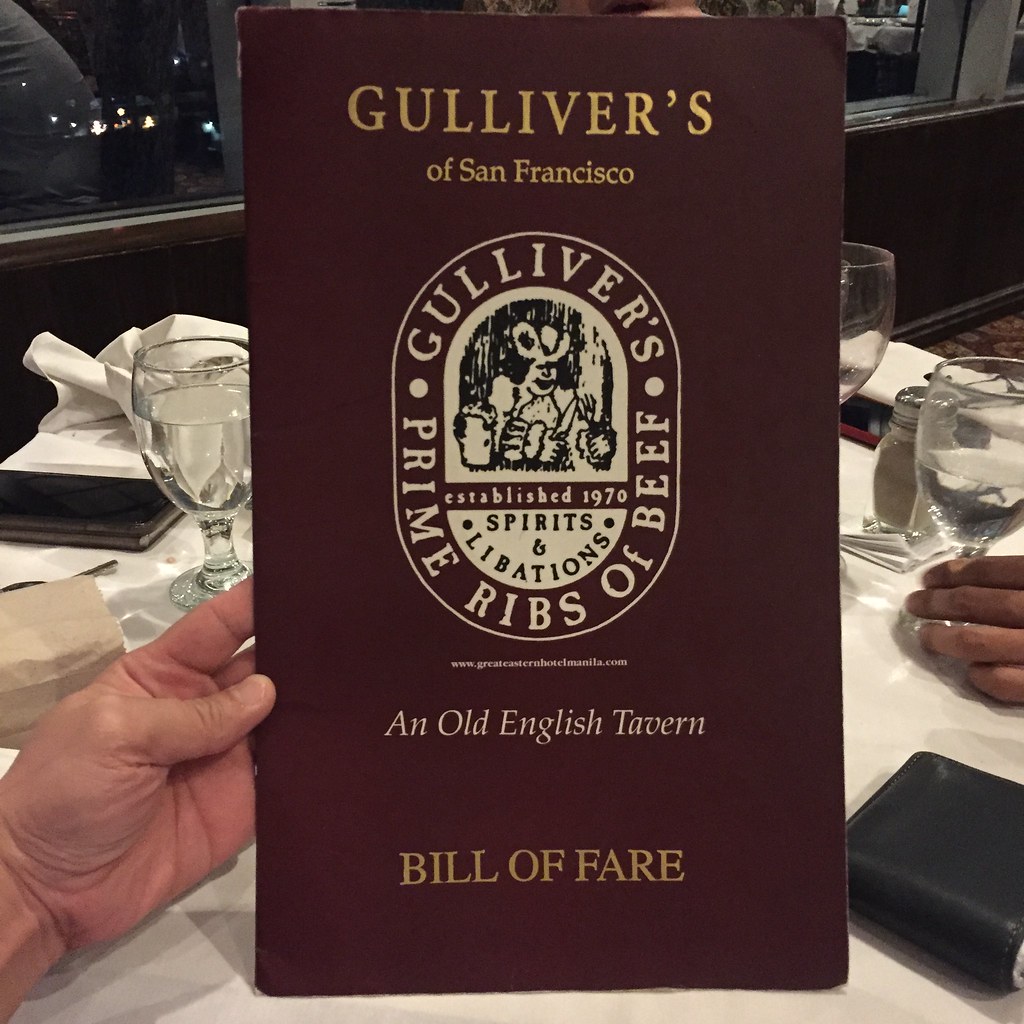The image depicts an old-school tavern's restaurant setting where patrons are seated at a dining table adorned with a white tablecloth, fine glasses filled with water or possibly wine, and napkins. In the center, a large maroon booklet, embellished with gold lettering, is being held by a person, possibly a white man judging by his hand. The booklet, resembling the size of a large magazine, reads "Gulliver's of San Francisco" at the top and "Bill of Fare" at the bottom, with phrases like "An Old English Tavern," "Prime Ribs of Beef," "Established 1970," and "Spirits and Libations" also inscribed. The cover art features a barmaid holding a beer alongside a man in a hat who is seated at a table with a fork, knife, and beer. The background reveals more details of the ambiance, such as a window with a visible wooden bottom, a brown carpet, and other diners' phones and hands resting on the table. A small black wallet is also seen adjacent to the menu.